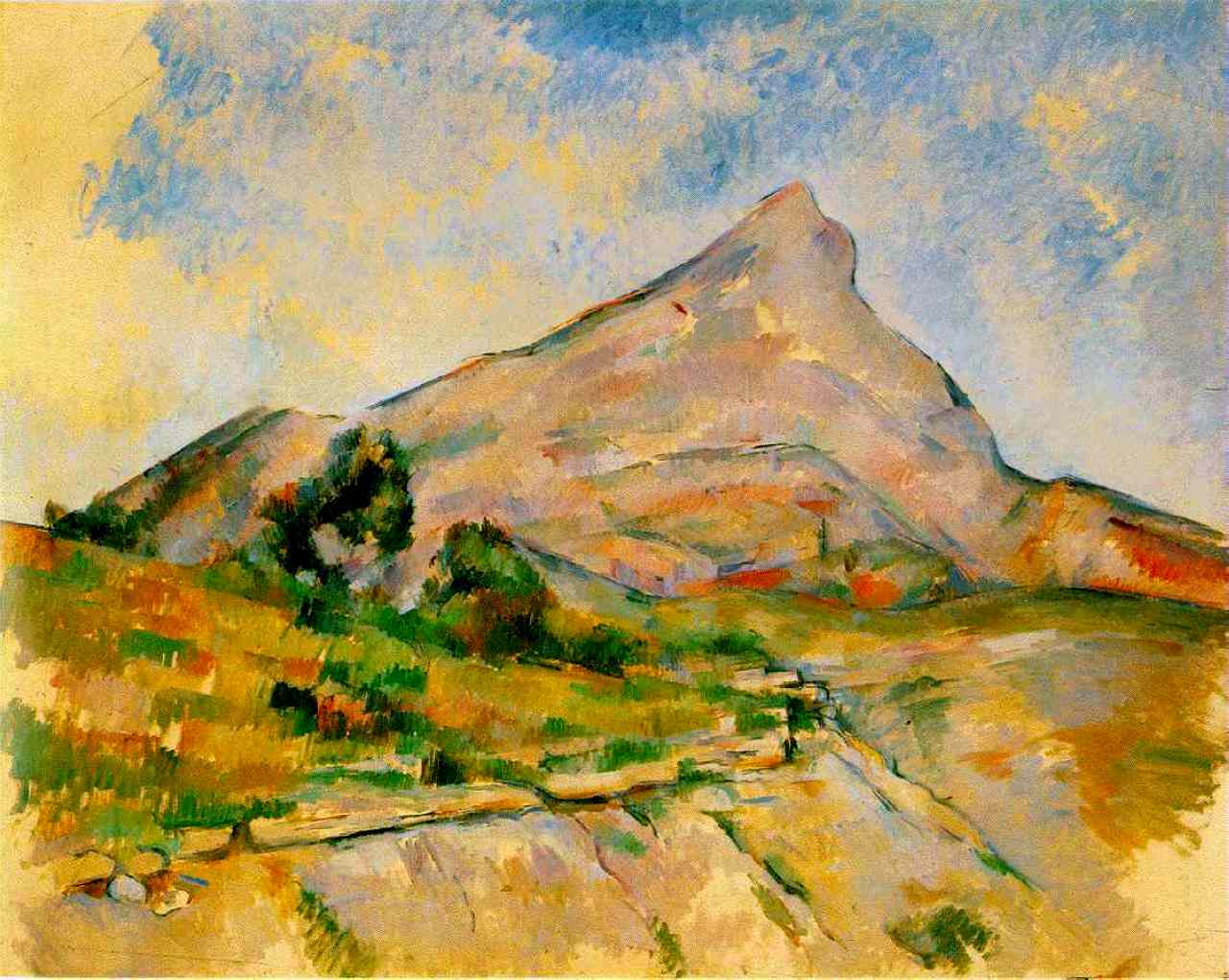This painting depicts a vibrant, impressionistic landscape featuring a majestic mountain that rises prominently from a sparsely vegetated valley. The scene is infused with a myriad of colors, presenting the mountain in varied shades of gray, orange, yellow, and a significant red streak on the lower right which could represent autumnal foliage. The valley in the foreground has patches of green grass, dirt, and rocky outcrops. Scattered bushes and shorter trees suggest a higher elevation or a semi-desert environment, and there is an overall sense that the landscape is not densely populated, perhaps making it ideal for camping. The sky is a stunning blend of blue and gold, enhancing the dynamic and colorful essence of the painting. There are no people or buildings in this scene, emphasizing the untouched, natural beauty of the landscape.